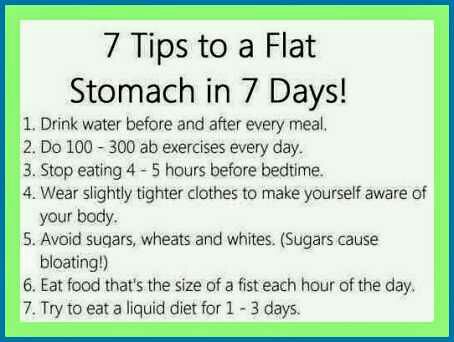The image is a slightly grainy, minimalistic poster with digital JPEG artifacts, seemingly pulled from the internet as a weight loss advertisement. It features a white background with a light green inner border and a dark green outer border. At the top, a bold heading in black text reads, "7 Tips to a Flat Stomach in 7 Days." Below the heading, the image lists seven numbered tips in black letters: 

1. Drink water before and after every meal.
2. Do 100 to 300 ab exercises every day.
3. Stop eating 4 to 5 hours before bedtime.
4. Wear slightly tighter clothes to make yourself aware of your body.
5. Avoid sugars, wheats, and whites. (Sugars cause bloating.)
6. Eat food that's the size of a fist each hour of the day.
7. Try to eat a liquid diet for 1 to 3 days.

The poster is straightforward with no additional imagery or graphical inclusions beyond the described text and borders.